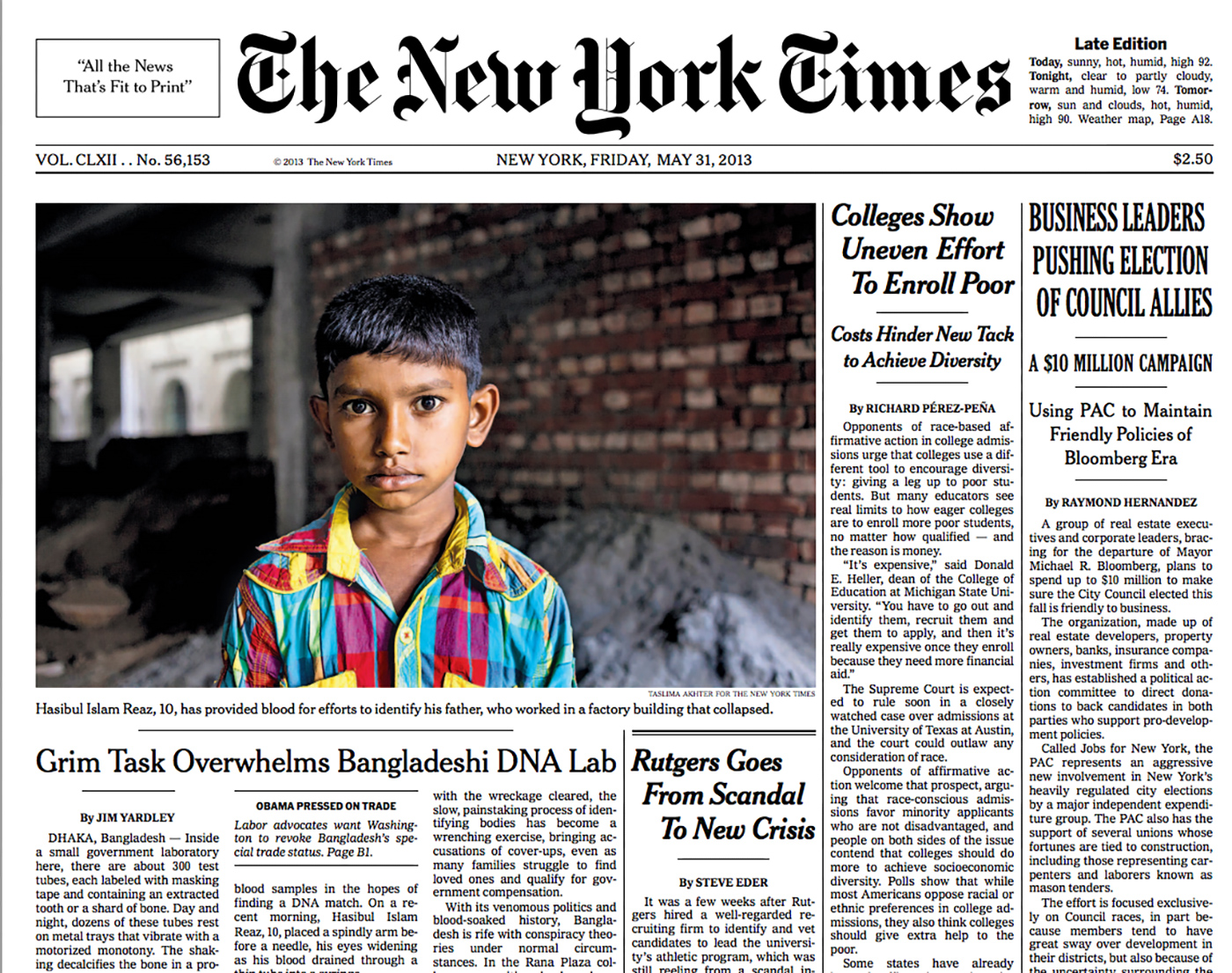The headline from the New York Times displayed in the image is from the late New York Friday edition, dated May 31st, 2013. The iconic New York Times masthead is present, alongside the famous slogan, "All the News That's Fit to Print." 

The main headline includes a prominent color photograph of Islam Reyes, a 10-year-old boy who provided a blood sample to help identify his father, a factory worker who perished when a building collapsed in Dhaka, Bangladesh. The headline accompanying the image reads, "Grim Task Overwhelms Bangladeshi DNA Lab," highlighting the overwhelming challenges faced by local authorities.

Adjacent to this story, another headline details turmoil within Rutgers University: "Rutgers Goes from Scandal to New Crisis." 

Additionally, the top section of the front page features two leading articles: "Colleges Show Uneven Effort to Enroll Poor," and "Business Leaders Pushing Election of Council Allies; A Ten Million Dollar Campaign."

The weather forecast for the day predicts sunny, hot, and humid conditions with a high of 92°F, followed by a clear to partly cloudy night with a low.

Overall, the headlines paint a grim picture, reflecting a series of distressing and controversial events on that day.